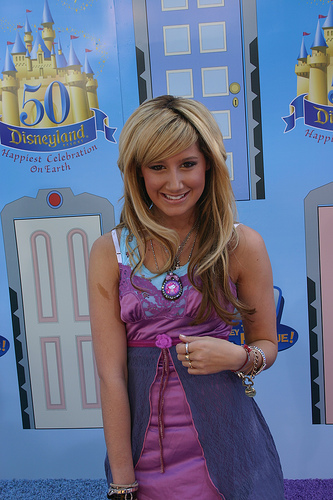In this image, a young lady stands at the center looking directly at the camera with a warm smile, displaying her top row of teeth. She has a distinct appearance with blonde hair on the sides and dark brown roots near her scalp, parted near the center and cascading down in front of her shoulders, covering her ears. Her skin is notably tan. She is dressed in a striking, sleeveless purple dress with an outer dark blue apron-like garment, revealing her shoulders and arms. Visible on her left shoulder is a brown mark. 

She accessorizes heavily, with numerous bracelets on both wrists, rings on her fingers, and a pendant featuring a cartoon girl logo around her neck. She holds one arm up in front of her stomach while the other arm hangs down naturally. Her costume is intricate, resembling those worn at cosplay events, complete with various patterns and designs.

In the background, a banner depicts a Disney theme with a blue door featuring grey sides and displaying the text "50 Disneyland" and "Happiest Celebration on Earth". Additionally, there is another door image in white with a red circle on top and a partially visible pink door. The setting appears to be indoors, possibly at an amusement or themed park like Disneyland, with a light blue, red, yellow, gray, pink, purple, and tan color scheme contributing to the lively atmosphere. The ground looks to be carpeted, adding to the indoor environment's cozy feel.